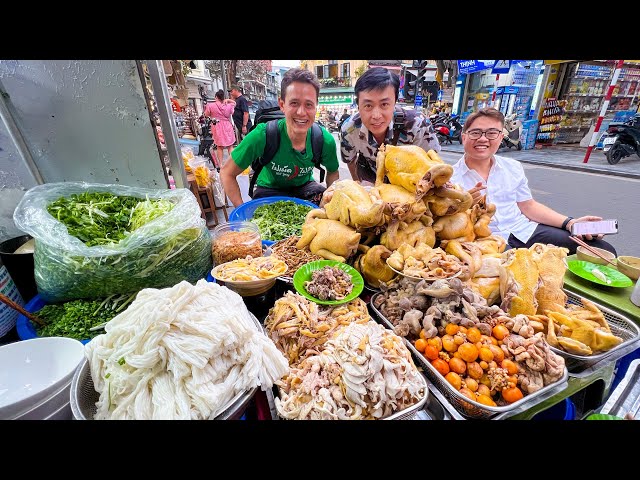In this vibrant street market scene, we see an outdoor food stand adorned with a wide array of colorful ethnic foods, including yellow and orange vegetables, and various types of chicken ready to be served with pre-made noodles. The food, likely intended for dishes such as pho, is placed in numerous bowls and plates, showcasing fresh mung beans, basil, cilantro, and other accompaniments. Against this lively backdrop, three men with Asian features are smiling directly at the camera, exuding a sense of joy and enthusiasm. One of them, standing on the right, is holding his phone, and another appears to have a backpack, suggesting they might be tourists capturing this culinary adventure. Behind them, the bustling street scene is illuminated under a bright, possibly partly cloudy sky, with buildings and shops displaying vibrant colors. The photograph, taken with a special wide-angle lens that slightly stretches the edges, encapsulates the lively and delightful atmosphere of this high-traffic street market.